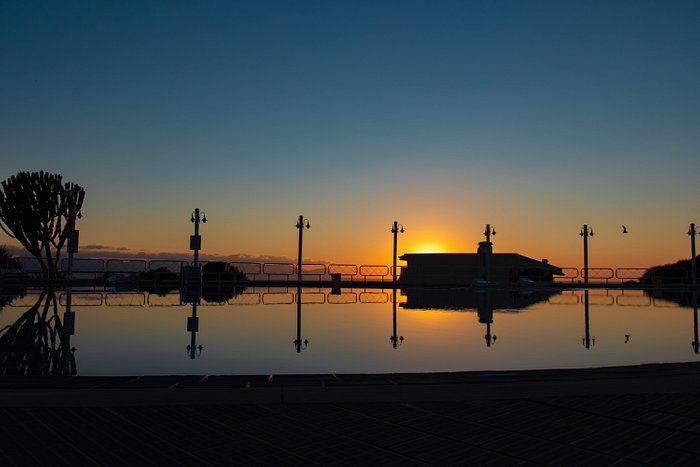The photograph captures a stunning outdoor sunset scene. The dark blue sky at the top transitions into a mesmerizing blend of yellow, orange, and red hues as the sun sets. In the foreground, the ground is dark, and a small body of water reflects the vibrant colors of the sunset. Emerging from the water are six light poles, each capped with a structure resembling a set of headphones. These poles are aligned along what appears to be a bridge. In the center of the image stands a dark, low building with a slanted roof and a chimney, casting its reflection into the water. On the left side, there is a silhouette of a tree and some bushes. A rectangular-shaped fence runs behind the building, further enhancing the depth of the scene.